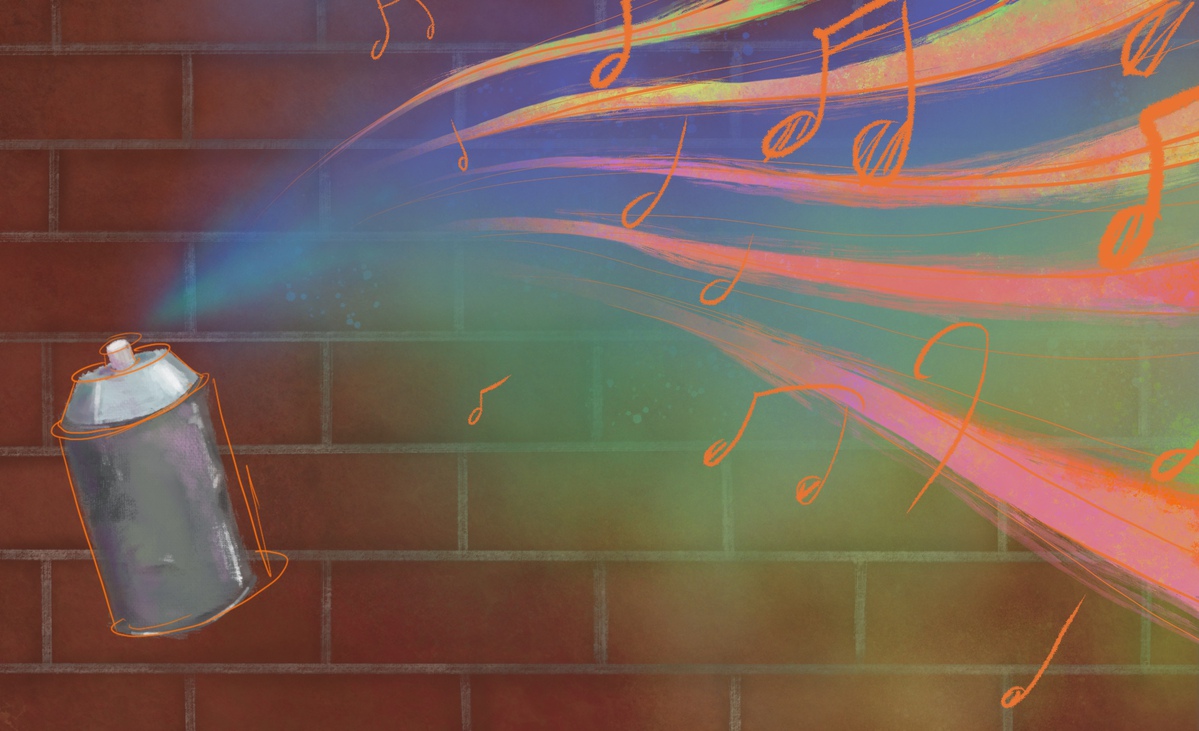The image is a vibrant, abstract artwork set against a red brick wall. The wall serves as the backdrop, with visible sections of exposed brick on the top and bottom left. Prominently featured is a spray paint can on the left side of the image, rendered in shades of gray with a white cap and outlined in a bright, fluorescent orange. The spray can appears suspended in the air, emitting a dynamic burst of colors including dark blue, light green, pink, orange, yellow, and neon green. These colors blend and spread outward, creating a lively, multicolored spray effect. Amidst this colorful spray, scattered across the right-hand side, are musical notes drawn in the same fluorescent orange, adding a whimsical element to the composition. The overall effect is energetic and playful, transforming the brick wall into a canvas of vibrant creativity and musical expression.